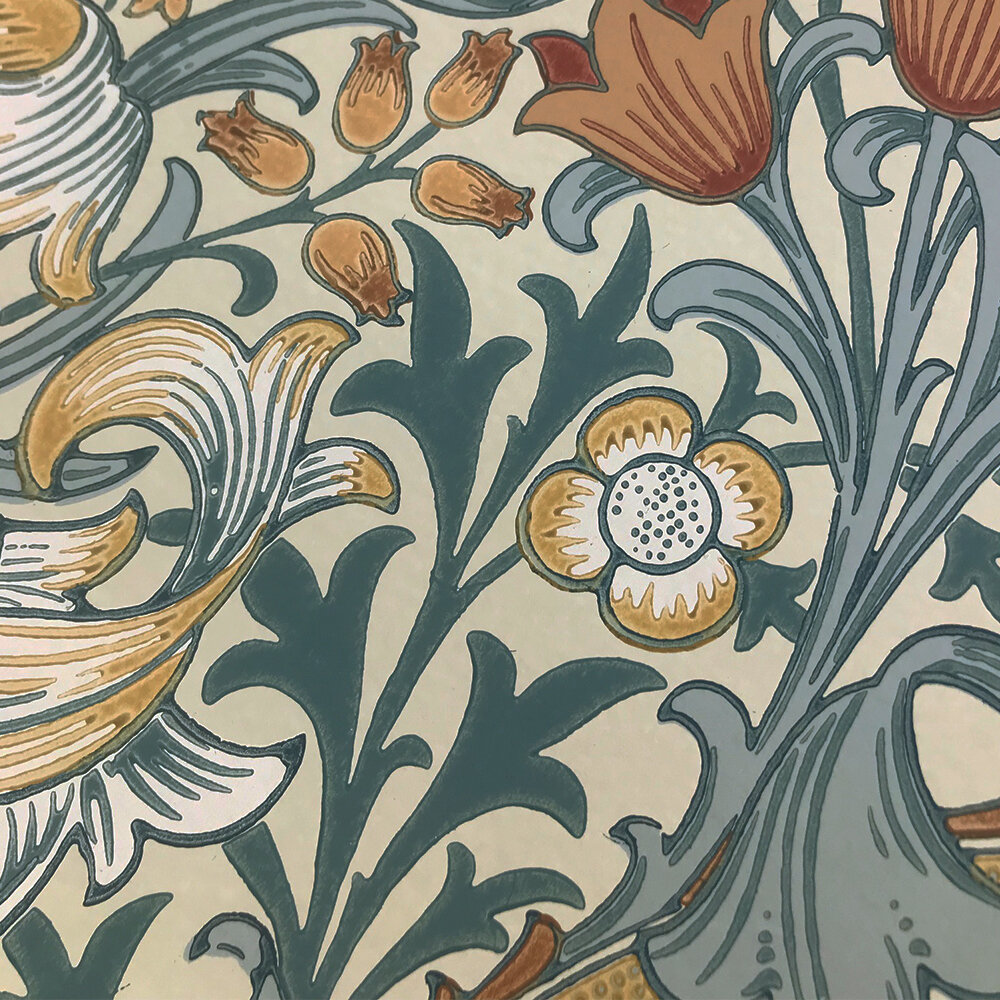The image captures a beautifully designed, possibly painted, floral wallpaper with a simple, yet intricate and unique style. The background is a light greenish-gray hue, providing a serene canvas for a plethora of flowers sprawling across the surface. Prominent in the design are four-leaf flowers in the center with intricate details, reminiscent of lilies with long, greenish-gray stems and leaves. Various flower types are depicted, including sunflower-like shapes, orange tulips with red-lined details, and clusters of lilies of the valley featuring tiny flowers on dark green stems. Some flowers display unopened buds, while light orange and white leaves interspersed with blue lines add delicate touches. The overall design conveys a sense of a sprawling garden, with flowers of various colors—yellow ochre, orange, and blue hues—harmonized in an almost whimsical, freeform arrangement that captivates the viewer's eye.